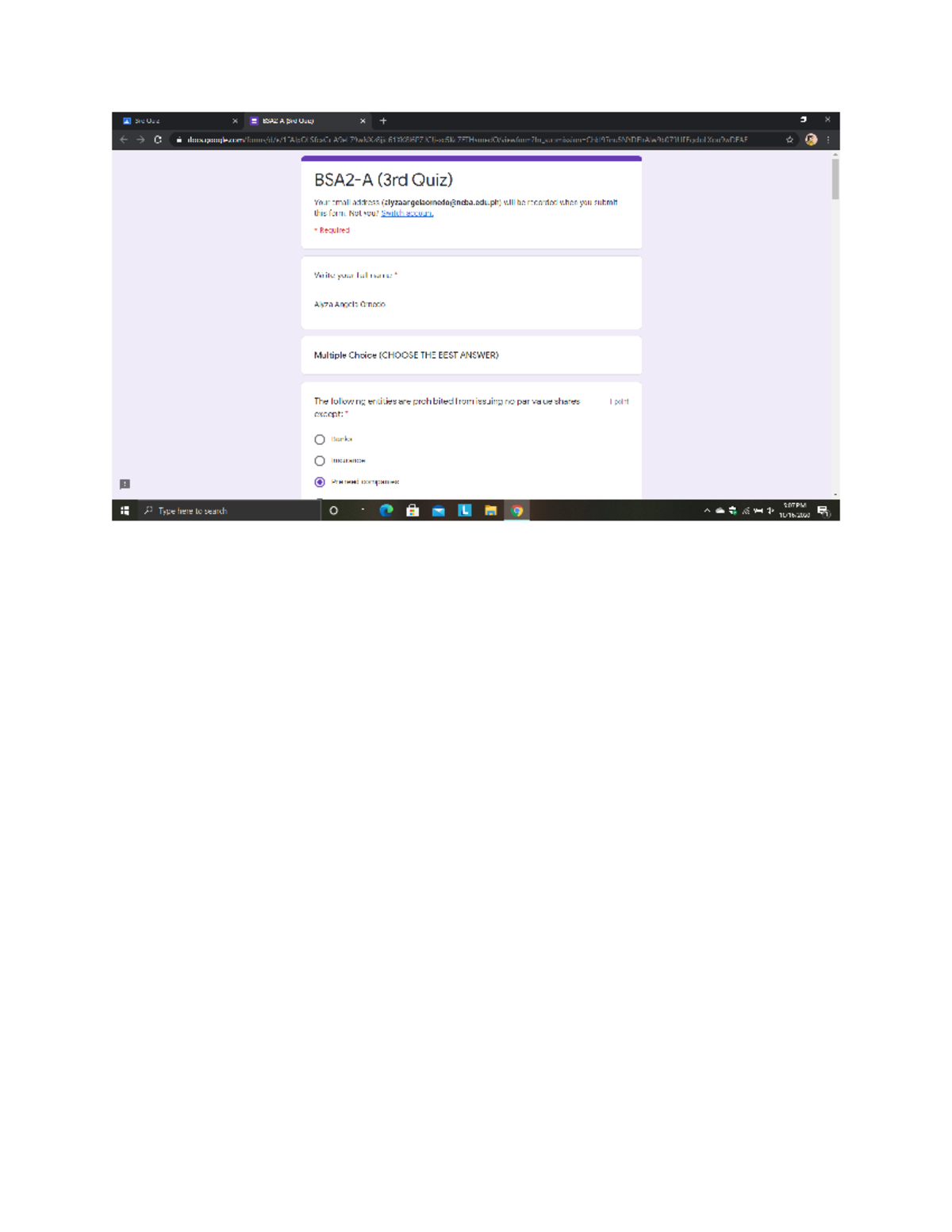**Caption for Screenshot of a Tabbed Browser in Google Forms Quiz**

The screenshot depicts an internet browser with multiple tabs open. The first tab on the left is partially blacked out with text that reads "third," though it is too small to discern completely. The second tab, which is selected, shows the title "BSA2-A third quiz" within brackets. The URL displayed starts with "docs.google.com/" followed by an unreadably long string.

The background of the webpage is pink and features a gray vertical scrollbar on the right. The header of the form is predominantly purple. The main text field reads "BSA2-A third quiz," followed by a notice indicating that your email address will be recorded upon form submission. There is an underlined blue text "Not used, but you count" and the phrase "This is required" marked with a red asterisk. An additional note clarifies that any field with an asterisk is mandatory.

Below this, there is a white input field labeled "Write your full name" with a red asterisk next to it. The entered name appears to be "Elisa Angelo Aredo" or something similar. Following this is a panel containing a multiple-choice question with an instruction to "Choose the best answer" written within brackets. The question underneath asks, "The following entities are prohibited from issuing no par value shares except" followed by an asterisk. The answer options listed are "Banks," "Insurance," "Preferred companies," with the last option truncated and unreadable. The option "Preferred companies" appears to be selected.

At the bottom of the screenshot, the Windows taskbar is visible. It includes the Windows logo on the far left, a search bar, several standard icons, and specific icons for a web browser, Play Store, email, Chrome, folders, and an unknown application marked with an "L." To the right side of the taskbar, there are additional icons, possibly for antivirus notifications, and the time displayed as 5:00 p.m., alongside other notification symbols.